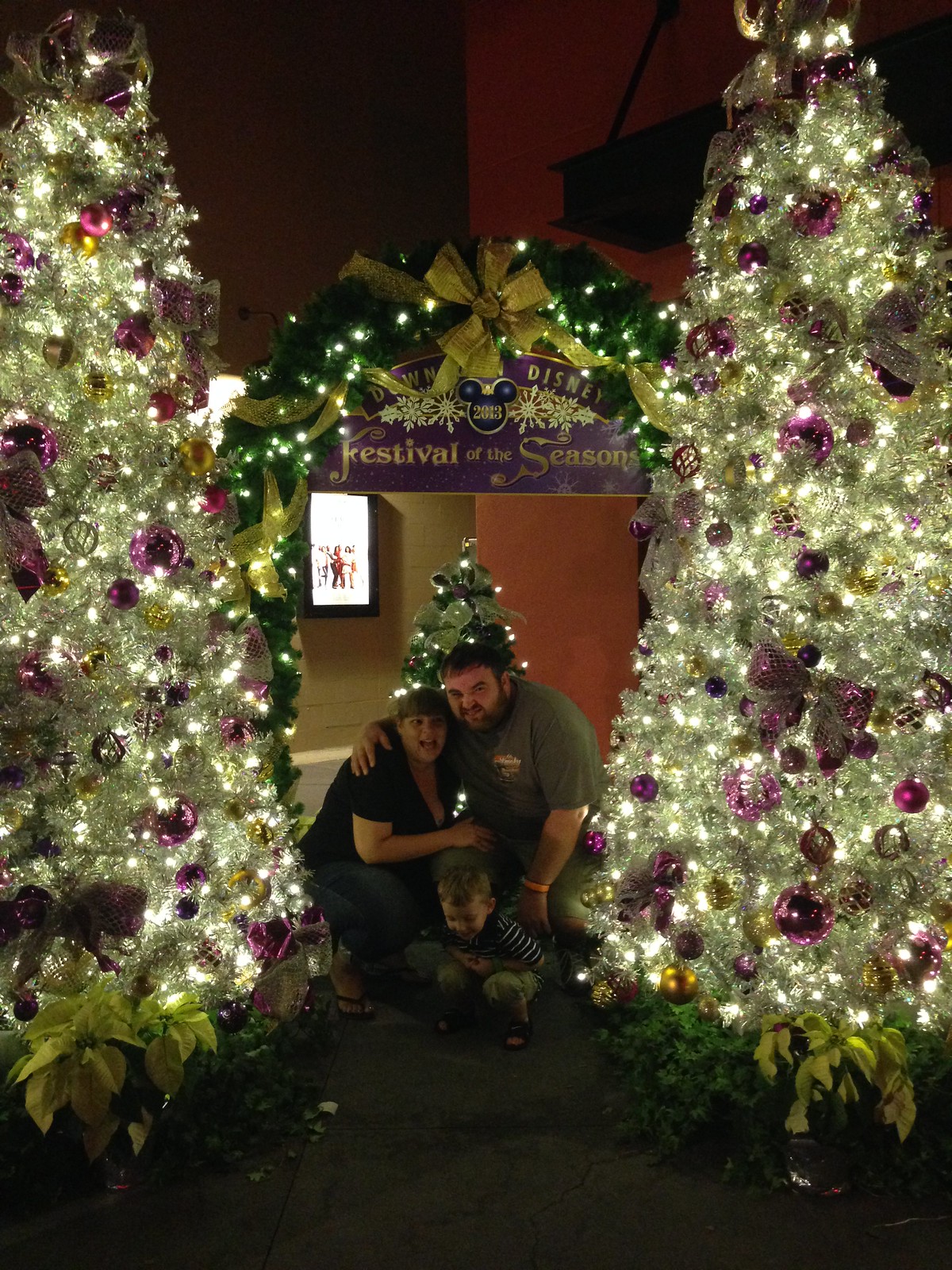The photograph, likely taken indoors at Downtown Disney in 2023, captures a Caucasian family—a husband, wife, and their young son—crouching between two beautifully lit Christmas trees adorned with white lights and embellished with purple and gold decorations, including silver balls and white bows. The husband, sporting a green shirt, shorts, and facial hair, has his arm around his wife, who is dressed in a short-sleeved black shirt, jeans, flip-flops, and a hat. Their son, dressed in sandals and a black and white striped shirt, kneels in front of them. Above the family, there's an archway decorated with garlands and lights, featuring a purple banner with gold lettering that reads "Festival of the Seasons, Downtown Disney 2023." The dark background accentuates the festive, well-lit scene, suggesting the photo was taken in the evening.